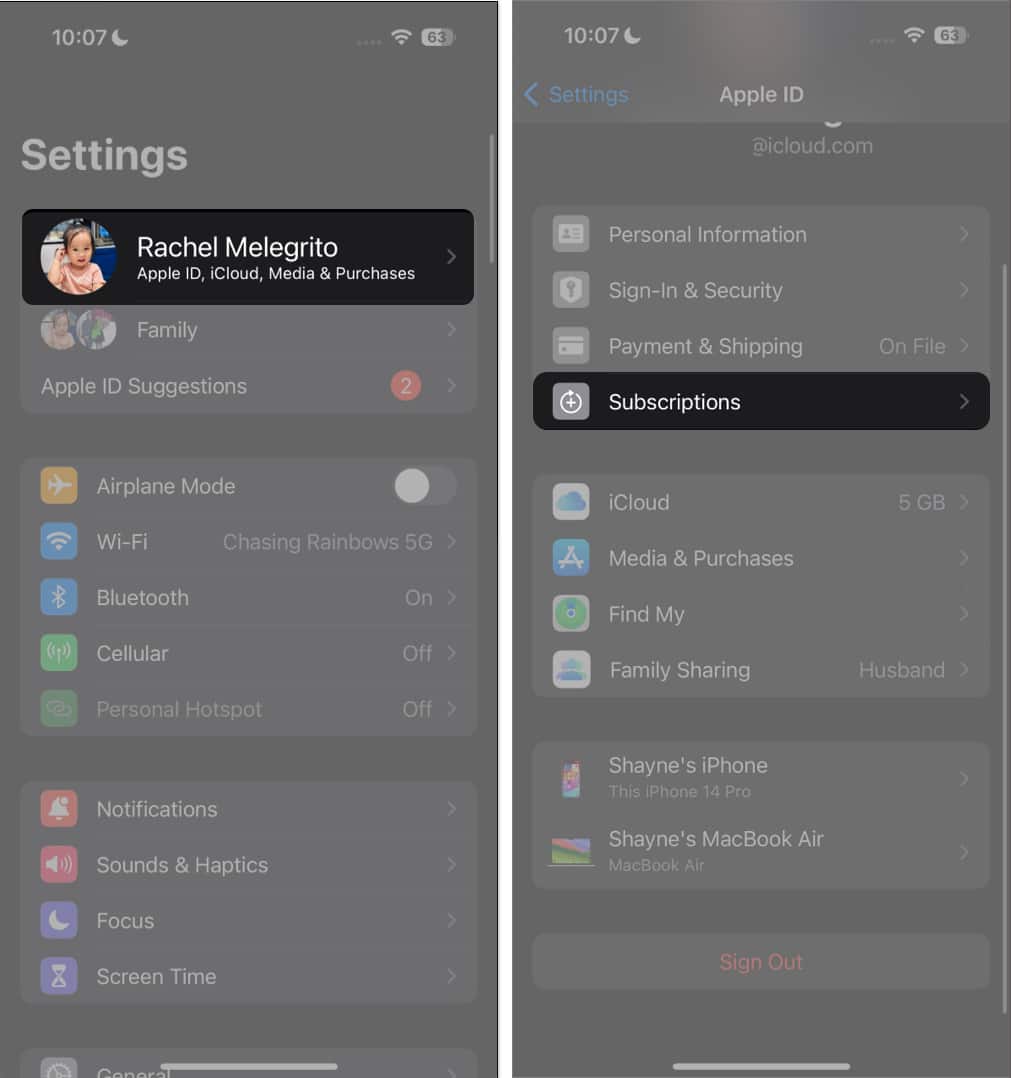The image consists of two side-by-side screenshots of an iPhone's settings interface. 

The screenshot on the left displays the home settings page, with the time reading '10:07' and a crescent moon icon indicating Do Not Disturb mode is active. The iPhone has no cellular signal but is connected to Wi-Fi, and the battery level is at 63%. The title "Settings" is at the top of this page, with a highlighted entry for "Rachel Malagrito" under "Apple ID, iCloud, Media & Purchases." The remaining options, including Family, Apple ID Suggestions, Airplane Mode, Wi-Fi, Bluetooth, Cellular, Personal Hotspot, Notifications, Sound & Haptics, Focus, and Screen Time, are all grayed out.

The screenshot on the right shows a detailed view of the Apple ID settings, beginning with a back arrow labeled "Settings" in blue at the top. Below, the list includes options such as Personal Information, Sign-in & Security, Payment & Shipping, Subscriptions, iCloud, Media & Purchases, Find My, Family Sharing, Shane's iPhone, Shane's MacBook Air, and Sign Out. In this screenshot, the "Subscriptions" option is highlighted in dark black, drawing attention to it while the other options are grayed out.

Combined, these screenshots illustrate the steps to check subscription statuses through the iPhone settings.